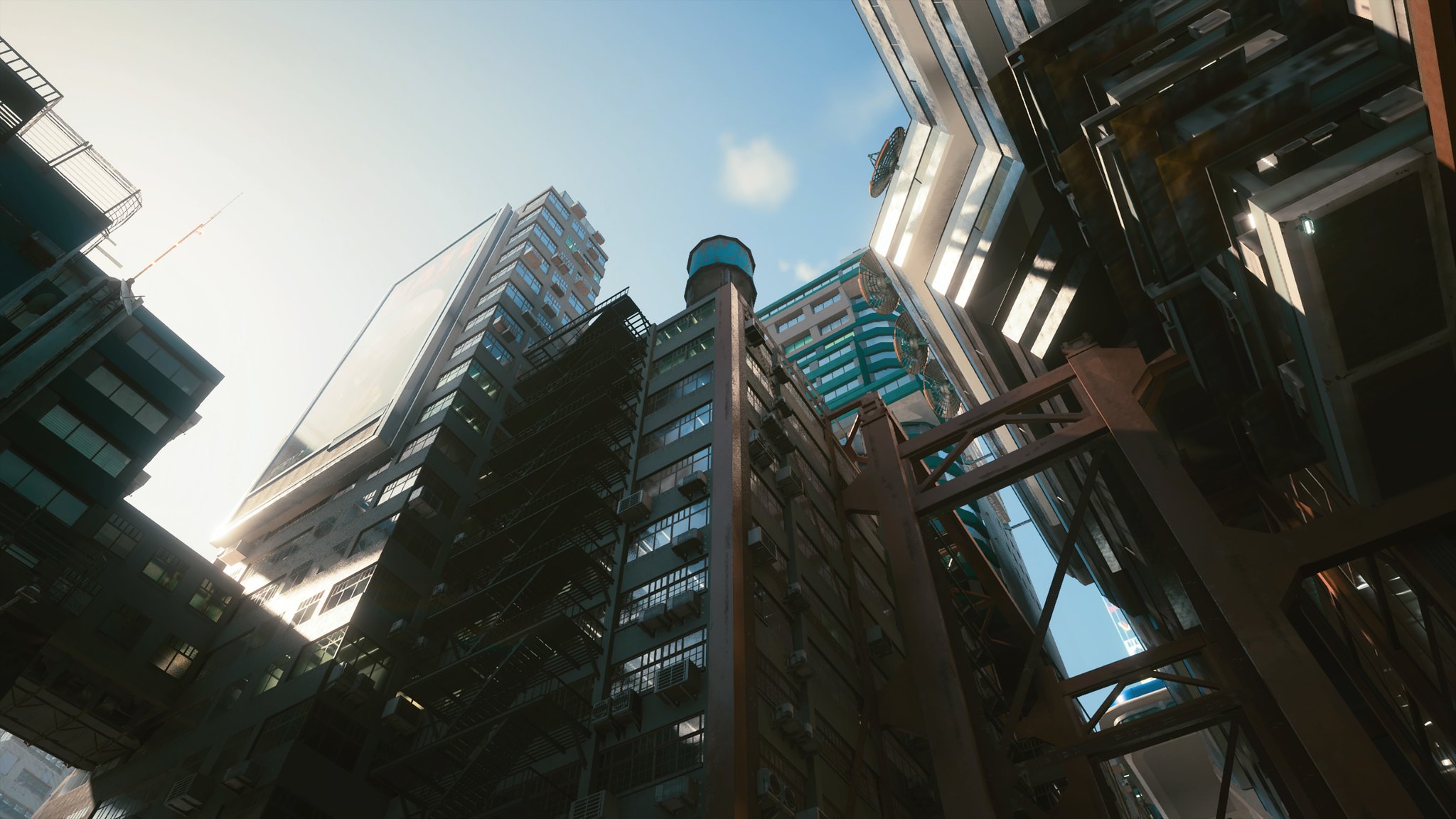This detailed image, seemingly a screenshot from the game Cyberpunk 2077, captures a dynamic and highly detailed view of a futuristic cityscape from street level. Dominating the scene are a pair of connected, rust-colored high-rise buildings, each towering at least ten stories. The buildings feature a modern design with numerous windows, defined balconies, and intricate white patterns against the brown facade. One building on the right showcases sharp angles and has notable exterior staircases akin to fire escapes, with a distinctive blue cylinder perched at one corner. The buildings are linked by massive steel beams, adding a layer of industrial strength to the architectural aesthetic. Rising from the courtyard between these structures is a metal tower intersecting both buildings, possibly for structural support.

To the left of the main buildings, there's an assortment of other high-rises, characterized by their bright blue windows and multiple balconies. A significant feature atop the right building is a large satellite dish, indicating the city's advanced technological setup. The skyline is further accentuated by a prominent, but blurry, billboard on the left and a vibrant blue sky filled with white, puffy clouds, providing a vivid backdrop to the urban landscape.